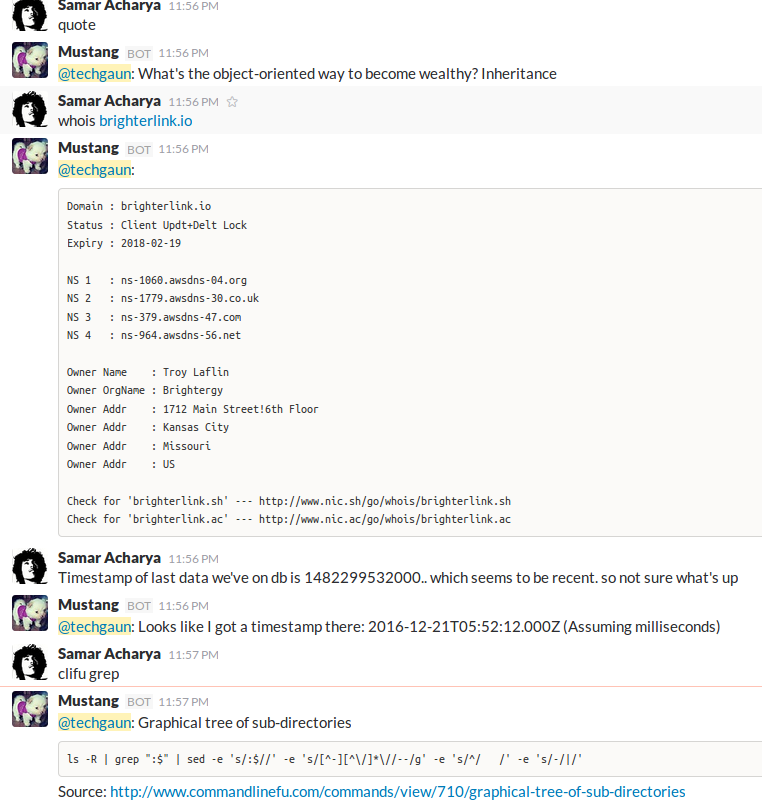Screenshot of an online conversation between Samar Akaria and Mustang discussing database information. The upper part of the screenshot shows their chat, where they talk about the data, beginning with details like "domain: writerlink.io", "status: client update + delete lock", and "expiration: 2018-12-19." Following this, there is a comprehensive block of data that seems to detail various parameters. The conversation continues below this data, with both individuals referring to and commenting on the database information displayed. The chat includes timestamps that show the sequence of their discussion. At the bottom of the screen, Mustang inputs what seems to be code for compiling a graphical tree of the subdirectory structure, and provides a source URL for where the information was obtained.